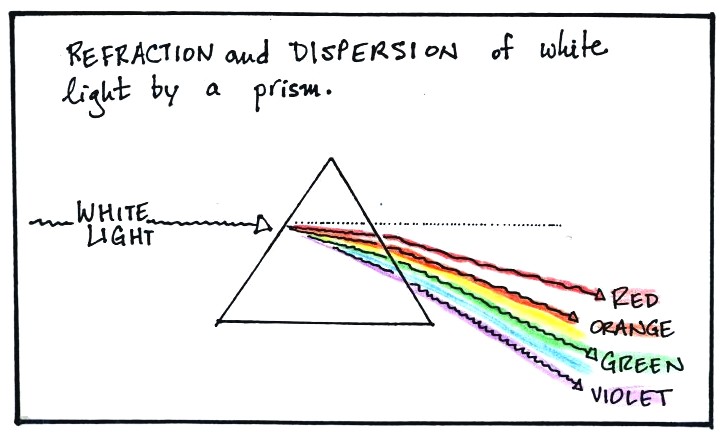The illustration depicts the scientific phenomenon of light refraction and dispersion through a prism. At the top of the image, handwritten in black ink, is the title "Refraction and Dispersion of White Light by a Prism." The central element is a black-outlined equilateral triangle, representing the prism, set against a white background. A black squiggly arrow on the left side indicates incoming white light, which strikes the prism. Upon hitting the prism, the light disperses into four distinct squiggly arrows, each colored respectively: red, orange, green, and violet. These arrows fan out towards the bottom right corner of the image, demonstrating the spectrum of light dispersed by the prism. A dotted horizontal line extends from the entry point of the white light, representing the original path and angle before dispersion. The entire diagram is bordered by a black rectangle, emphasizing its scientific context.